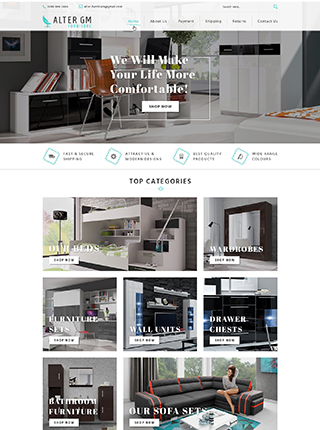The image depicts a screenshot taken from a phone of the Alter GM website, characterized by its tall, narrow rectangular shape. At the top of the screenshot, the website's name, "Alter GM," is prominently displayed. A hand icon is pointing towards the first menu option on the left, suggesting possible interactivity with the menu. The options in the menu bar include "About Us," "Payments," "Shopping," and "Contact Us."

The central part of the image features a somewhat blurry photograph of a well-decorated living room. Notable items in the living room include shelves, stands, cupboards, and a designated computer area with a brown chair slightly pulled out from the desk. Overlaid text in the middle of the image proclaims, "We will make your life more comfortable!" followed by an invitation to "Shop Online."

As the viewer's eye moves further down the image, there is a section showcasing various top categories of products available on the website. These categories include "Beds," "Wardrobes," "Furniture Sets," "Wall Units," "Drawer Chests," "Bathroom Furniture," and "Sofa Sets."